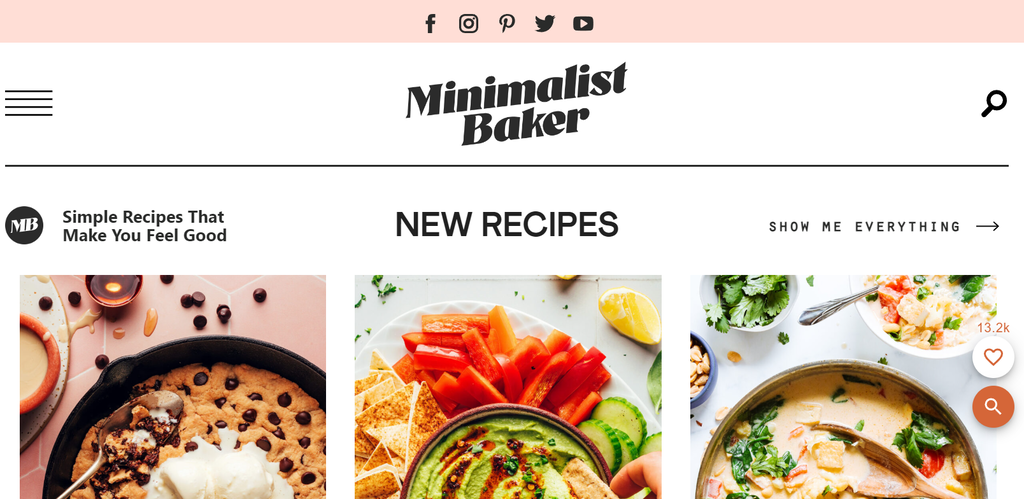At the top of the image is a pink rectangle featuring social media icons for Facebook, Instagram, Pinterest, Twitter, and YouTube. Directly beneath this, in slanted black bold letters, is the text "Minimalist Baker," accompanied by a search icon to its right. A thin black line runs underneath the text. On the top left corner, there are four horizontal lines stacked vertically, and below them, the initials "MB" appear with the tagline "Simple Recipes That Make You Feel Good." To the right of this section, in large bold black letters, it reads "New Recipes," and adjacent to that, another bold text states "Show Me Everything" with an arrow pointing to the right. 

Below this textual information, on the left side, is an image of a cast iron skillet cookie studded with chocolate chips. To its right is another image showcasing guacamole paired with tortilla chips, carrot slices, what appears to be either squash or cucumber slices, and lemon wedges. Further to the right is a final image depicting a creamy Alfredo dish.